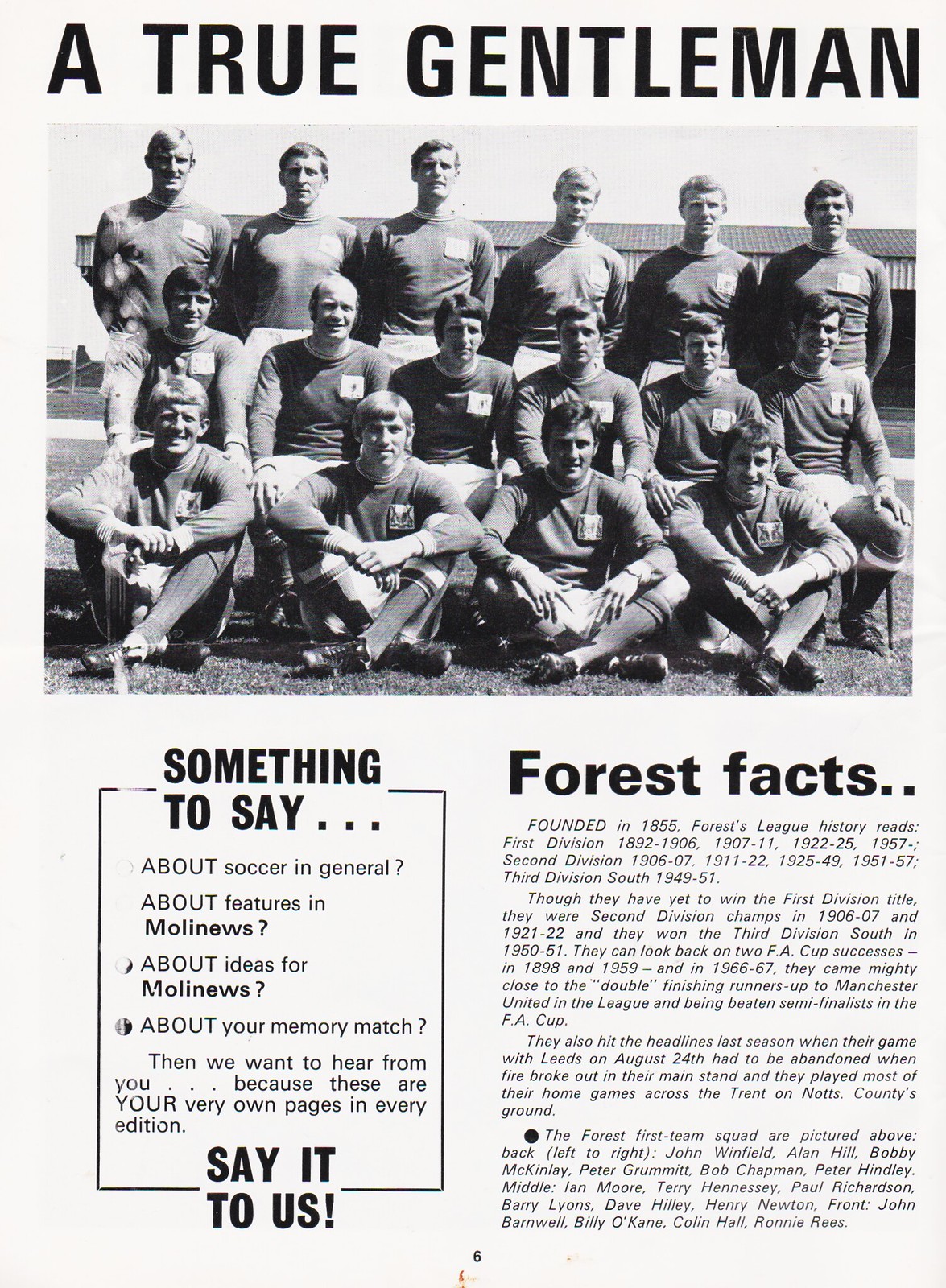This is a tall rectangular scan of a page from an old sports magazine, slightly off-white in color. At the top of the page, in bold black capital letters, it reads "A True Gentleman." Below this heading is a large black-and-white photograph of a soccer team posing in three rows. The back row consists of six men standing; the middle row has six men seated on chairs; and the front row features four men sitting on the ground. The players are all dressed in sporting uniforms, complete with shorts, high socks, and long-sleeved tops, each adorned with a square patch on the left breast.

Below the photograph, the page is divided into two columns. The left column features a tall rectangular box with bold text that reads "Something to Say..." followed by smaller text asking for input on various topics: "about soccer in general? about features in Molyneux? about ideas for Molyneux? about your memory match?" It concludes with an invitation: "Then we want to hear from you... because these are your very own pages in every edition. Say it to us!"

The right column is titled "Forest Facts" in large black letters, followed by a detailed history of the Nottingham Forest Football Club. This section outlines the club's league history, notable achievements including two FA Cup victories in 1898 and 1959, and a dramatic incident from the previous season when a game had to be abandoned due to a fire. The text also lists the names of the players in the photograph: Back row (from left to right): John Winfield, Alan Hill, Bobby McKinlay, Peter Grummitt, Bob Chapman, Peter Hindley. Middle row: Ian Moore, Terry Hennessy, Paul Richardson, Barry Lyons, Dave Hilly, Henry Newton. Front row: John Barnwell, Billy O'Kane, Colin Hall, Ronnie Rees.